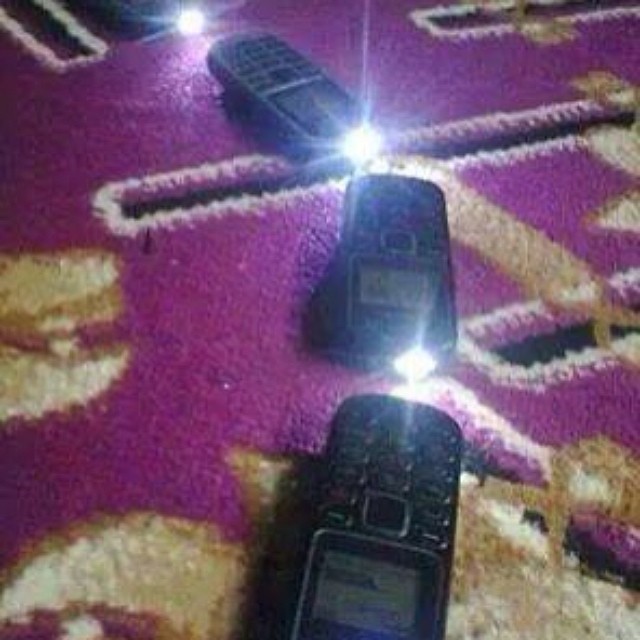The image depicts a line of four old-fashioned, black brick Nokia cell phones, each equipped with a keypad and a small rectangular black-and-white screen. These phones are arranged in a single file with a slight curve to the right, placed on a purple carpet or blanket that is adorned with intricate brown and gold patterns, including a few triangles with black centers and white trim. Three of the phones have their top flashlights on, casting a soft glow. The first phone, at the top of the line, has only its lit-up top visible. The second phone, slightly right and lower, displays its front but is out of focus. The third phone is positioned vertically, and though its details are blurry, the flashlight at the top is noticeable. The last phone at the bottom of the arrangement extends off the edge of the image with its flashlight out of view.